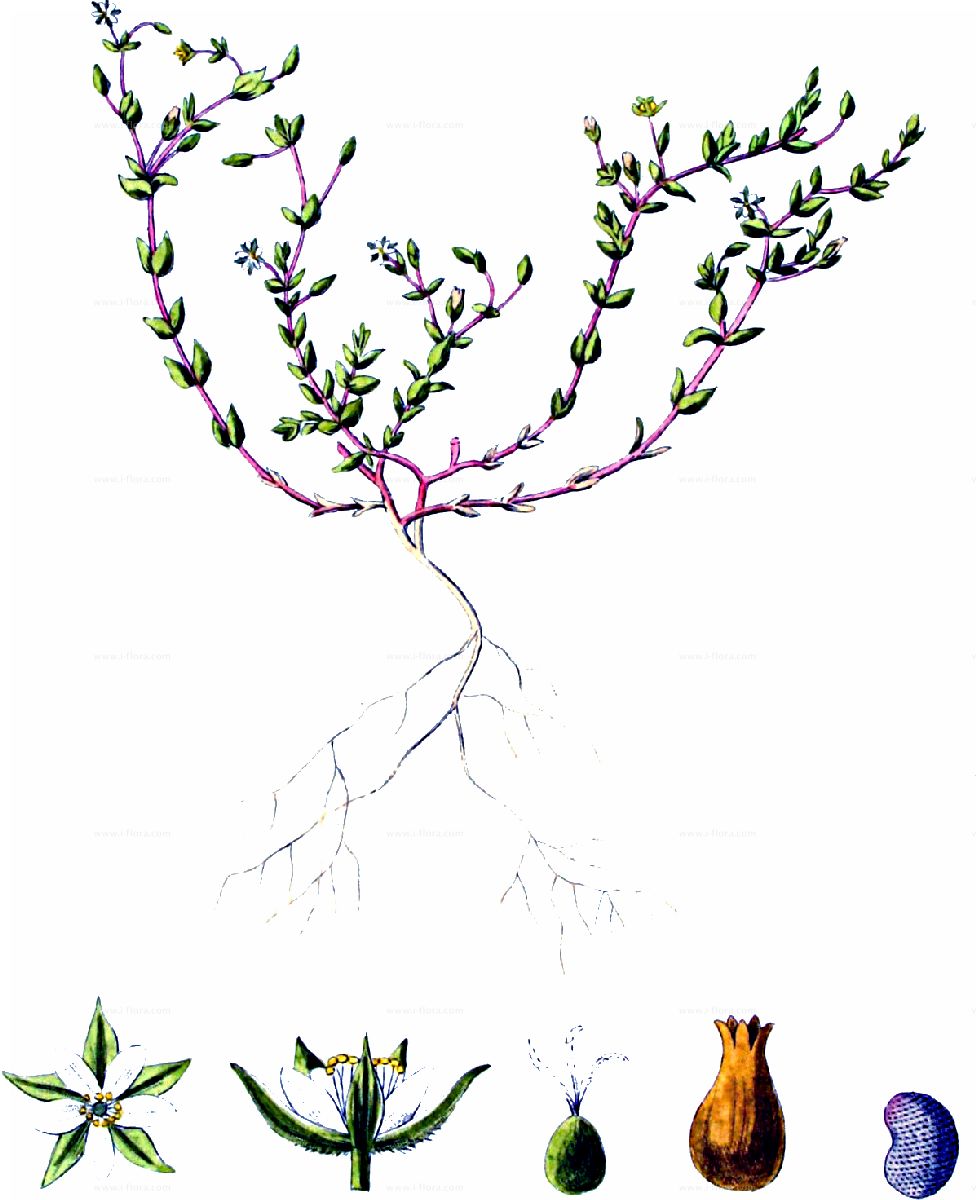The image depicts a detailed botanical illustration of a plant's growth stages, presented on a white background without any textual labels. At the top, a fully grown vine plant is intricately illustrated, featuring red stems, green leaves positioned opposite each other on the twigs, and tiny white flowers with blue centers and yellow stigmas. The plant's comprehensive structure is depicted, showing off the branches, leaves, roots, and budded flowers. The roots extend prominently from the base, showcasing several offshoot roots.

Descending from this, the illustration provides a sequential breakdown of the plant's growth phases. Starting from the left, the first image shows a top-down view of the leaves with a blue-centered flower. The second phase is a cross-sectional view of the similar flower, portraying the detailed positioning of the leaves, petals, and stigma. Next, the illustration depicts a fertilized flower that is beginning to swell. Following this, a brown seed capsule is shown, representing the mature seeded phase. The final image on the right presents a bluish bean, resembling a kidney bean, that signifies the last stage of seed development.

Overall, the comprehensive nature of this botanical plate offers an insightful depiction of a plant's lifecycle, from initial budding to full bloom and seed formation.